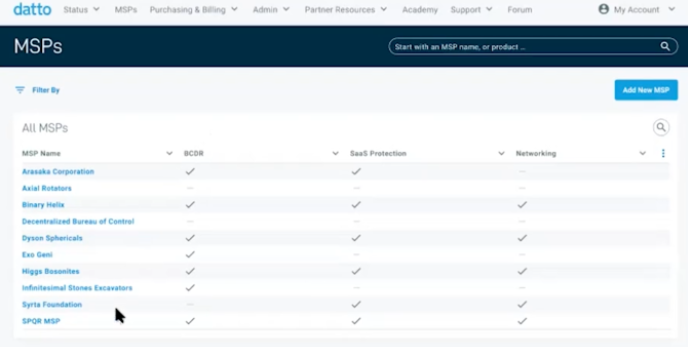The image is a detailed screenshot of the Datto website's user interface. At the very top, the word "Datto" appears in lowercase blue letters. To the right of it, black or gray text includes dropdown options labeled Status, SPS (Purchasing and Billing), Admin, Partner Resources, Academy, Support, and Forum.

On the right side of the top bar, there is a white person icon inside a black circle, next to the text "My Account" with an arrow indicating a dropdown menu. Below this top bar, against a dark blue or black background, the letters "MSP" are prominently displayed, with a lowercase "s". To the right, there's a search icon next to the text "Start with an MSP", followed by a magnifying glass icon.

Underneath this section, against a white background, there is a blue "Filter By" label with an icon of three horizontal lines of varying lengths. To the right is a blue button labeled "Add New MSP" in white text.

Below this, the heading "All MSPs" is in bold black font, followed by a smaller font with "MSP Name", which also has an arrow for sorting. Further down are headers like "BCDR" (in black capital letters), "SAAS Protection" (with what appears to be dollar signs or S's, and an arrow), and "Networking" accompanied by three blue dots.

The table lists various organizations and their corresponding statuses under each header:

- Arkansas Corporation: Checkmarks under BCDR and SAAS Protection, a dash under Networking.
- Axial Rotators: Dashes under all categories.
- Binary Helix: Checkmarks under all categories.
- Decentralized Bureau of Control: Dashes under all categories.
- Dyson Sphericals: Checkmarks under all categories.
- XOG: Checkmarks under BCDR and SAAS Protection, dashes under Networking.
- Higgs Benzenite: Checkmarks under all categories (the text is a bit blurry).
- Infestinal Stones Excavators: A checkmark under BCDR, dashes under other categories.
- Syria Foundation: A dash under BCDR, checkmarks under SAAS Protection and Networking.
- SPQR MSP: Checkmarks under all categories.

This table is set against a light gray background, with the text entries displayed on a white background.